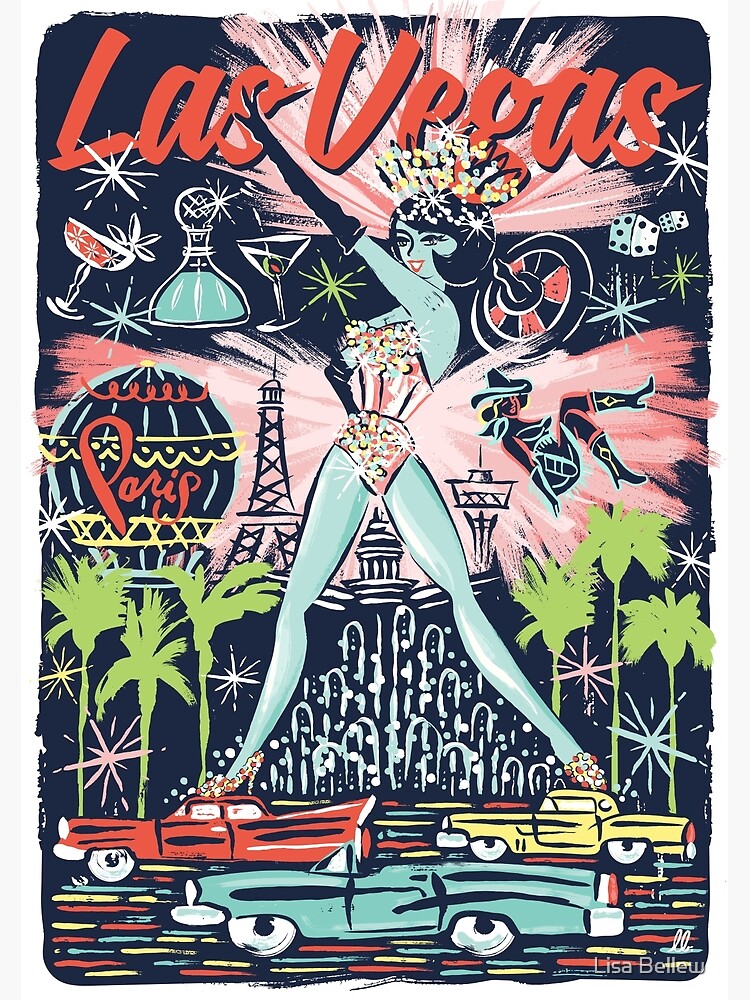This poster-style illustration of Las Vegas, evocative of a vintage graphic from the 1950s or early 1960s, features a prominent showgirl at its center. She has light blue, almost aqua skin and is adorned in a frilly pink sequin corset, complemented by a sparkling headdress and long black gloves. The showgirl strikes a confident pose with one hand on her hip and the other pointing upward, her short black bob accentuating her glamorous look. Surrounding her are various Las Vegas icons, including martini glasses, alcohol bottles, dice, and a roulette wheel, all depicted in a bold, simplistic brushstroke style akin to chalk drawings.

The background is dominated by a dark navy blue, almost black, hue that contrasts with subtle accents of green, pink, and white. At the top, the phrase "Las Vegas" is written in red cursive, while pink explosion lines and scattered stars add to the dynamic composition. In the backdrop, elements such as a tiny black Eiffel Tower, a "Paris" balloon, neon cowgirl sign, and palm trees enhance the scene’s cityscape. Towards the bottom, three vintage convertible cars—colored in red, teal, and yellow—drive past a grand fountain, reinforcing the image’s nostalgic feel. The entire illustration is encased in a somewhat grungy border, and a watermark at the bottom credits the artwork to Lisa Bellew.